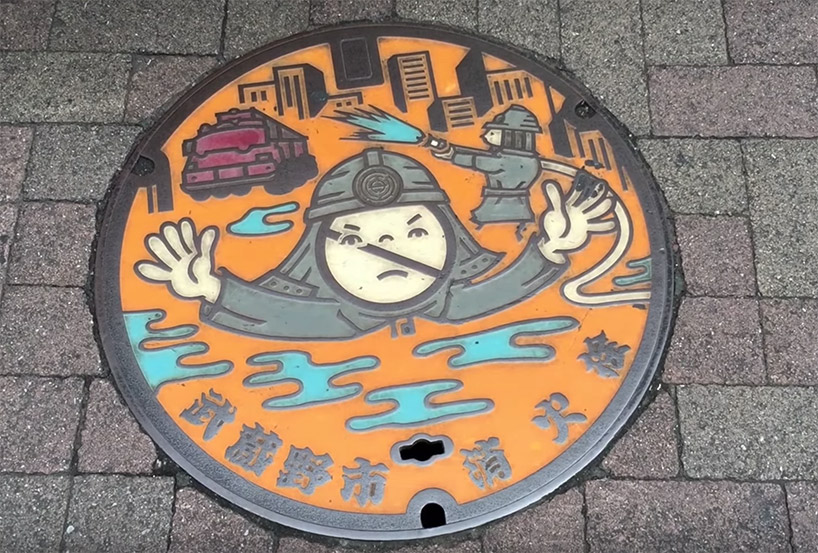This overhead photograph captures a vividly painted steel manhole cover set into a pebbly grayish dark blue brick pavement. The manhole cover features a bright yellow-orange background, prominently displaying a cartoonish figure at its center with a frowning expression, wearing a gray helmet and sleeves, and a circle-slash symbol over its face. Above this central figure, a scene unfolds with another character in gray firefighting gear, holding a hose amidst a backdrop of buildings and a fire truck. Piles of water, artistically shaped like curves, add dynamic elements to the scene. Japanese characters are inscribed around the bottom rim, identifying the city and noting "fire hydrant." The square paved surface's intricate details and the colorful, creative depiction make this manhole cover a striking piece of urban art.